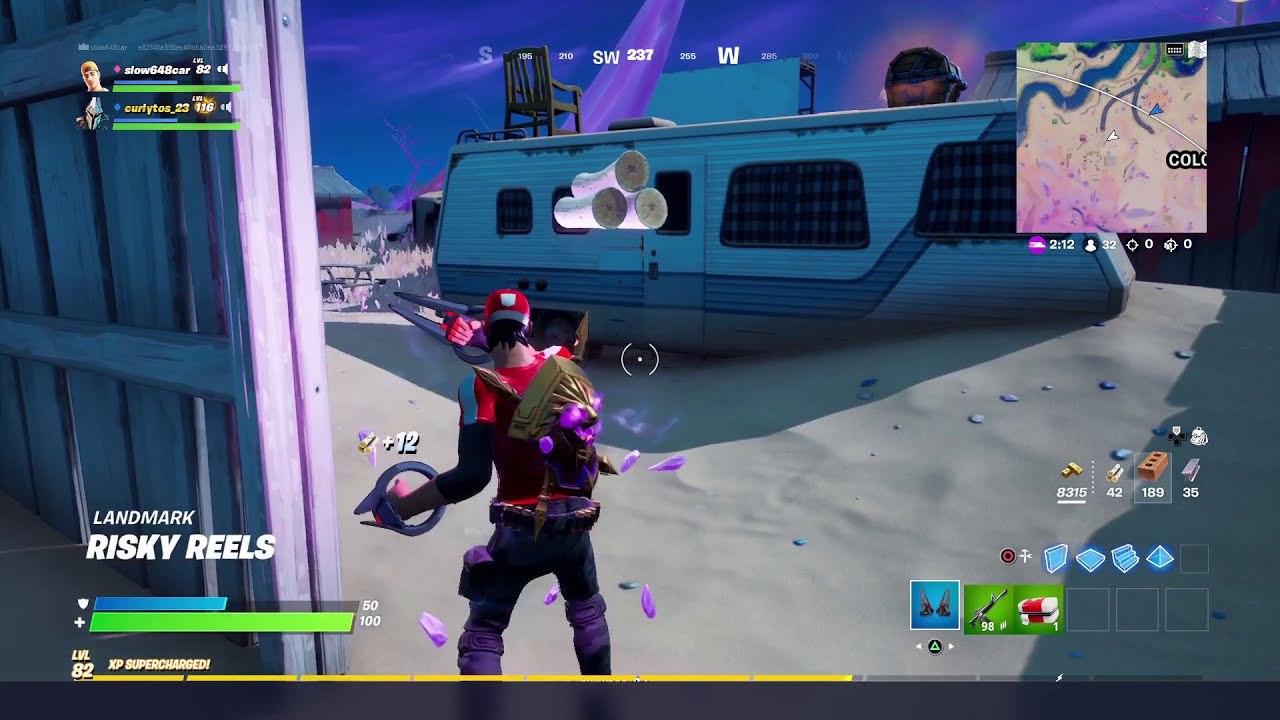This is a detailed screenshot from the video game Fortnite, depicting a scene in a sandy environment marked by a mobile home or RV with a chest on top. The primary focus is a character positioned near the bottom center of the image, clad in a red, black, and white outfit with jeans, and carrying a distinctive golden backpack featuring a lion's face with purple eyes. The visual is predominantly colored in shades of blue, gray, and red, with additional hues of pink, purple, green, and black scattered throughout. 

To the upper left, the character's active teammates are displayed, with one clearly named "CurlyToes_23." In the bottom left corner, the text "Landmark Risky Reels" indicates the location within the game. The character's health and shield bars are also visible here, showing a fully filled health bar and a half-full shield bar. There's a yellow experience bar indicating a level progression, noted as level 82 with supercharged XP. Additional on-screen elements include item counts, possibly currencies or resources, one of which is priced at $1.89. The overall layout, showcasing different health bars, buttons, and building materials, reinforces the game's interactive environment, suggesting the character is equipped and ready for action within this computer-generated landscape.